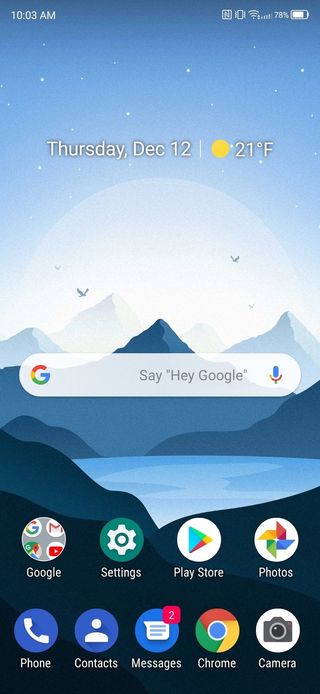The screenshot captures the home screen of a smartphone. The wallpaper features a serene landscape of mountains surrounding a lake, with a full moon in the background and a couple of birds in flight. At the top of the screen, it displays the time as 10:30 AM, with indicators for Wi-Fi connectivity and a battery level at 78%. The date is shown as Thursday, December 12th, and the weather is noted to be 21 degrees Fahrenheit and sunny.

Midway down the screen is a search bar with the text "Say Hey Google" and a microphone icon for voice commands. Below this are several app icons, starting with a Google folder that includes Chrome, Maps, YouTube, and Gmail. To the right of the folder is the Settings app, used for updating and configuring the phone. Next is the Google Play Store, identifiable by its green, red, and yellow triangle icon, followed by the Photos app, represented by a pinwheel in green, red, blue, and yellow.

On the bottom row of the screen, there are quick-access icons for Phone (a white phone on a blue background), Contacts (a white person silhouette on a blue background), Messages (with two unread messages), Google Chrome, and the Camera app, which provides direct access to the phone's camera function.